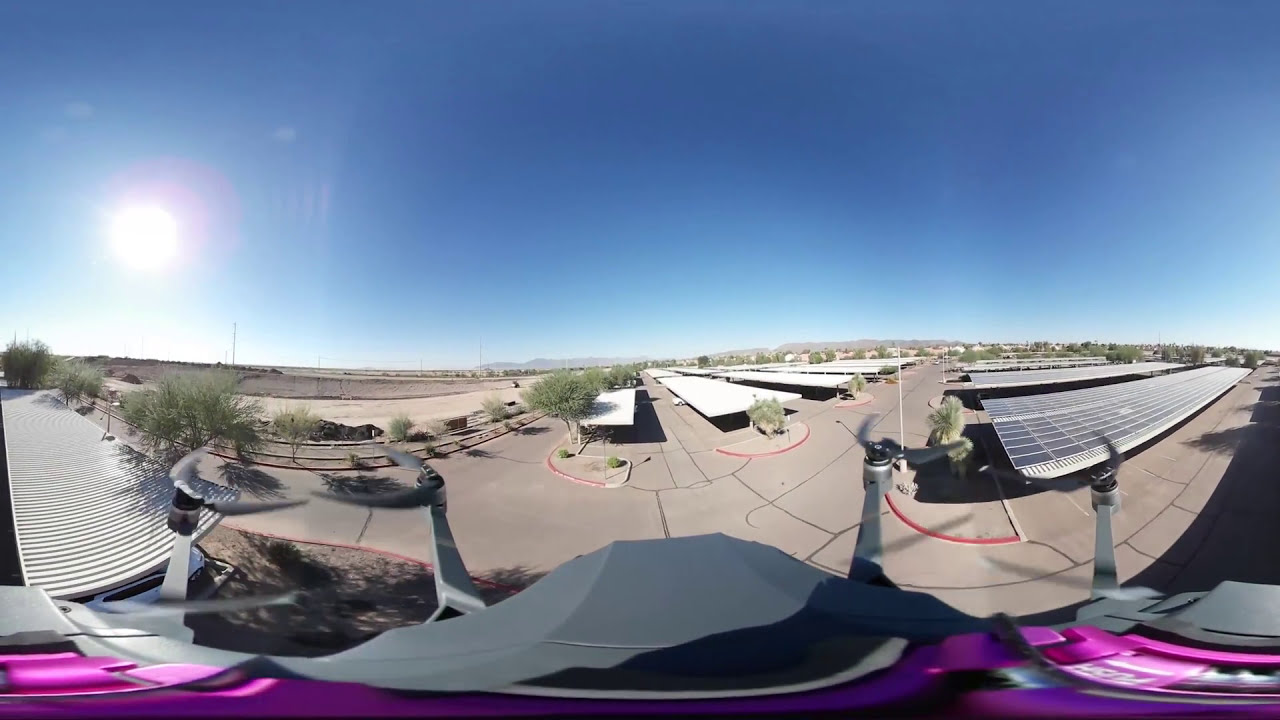This photograph, captured with an unusual lens and taken from above, likely by a drone, depicts an industrial or small airport area. The image showcases a diverse scene: in the foreground, the edges of the drone are visible alongside the hood of a vehicle, possibly a truck, flanked by purple areas. The bottom right features a tan-brown concrete parking lot accented by red curbs, with solar panels - bluish-white in color - installed on a nearby structure, hinting at a sustainable energy setup. To the right and throughout, modern low-lying white buildings stretch uphill, their appearance slightly distorted by the lens curvature, with a few trees interspersed and scattered cars. The left side is dominated by a corrugated material running parallel, and an open dirt lot extends to the far left of the image. Above it all, a clear blue sky encompasses the top half of the photograph, with the sun emitting a white glow from the far left. The overall hue of the scene blends earthy pinks, greens, and blues, emphasizing a mix of natural and industrial elements.